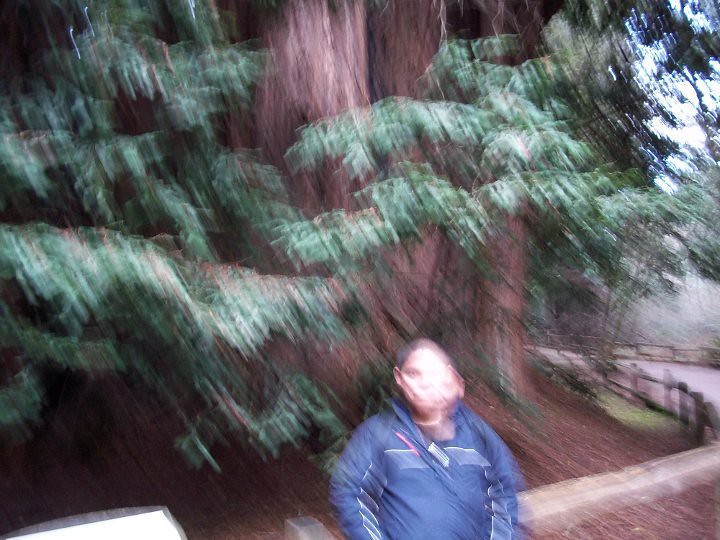This outdoor photograph is notably blurry and out of focus, capturing a scene in front of a substantial tree, possibly a redwood, with a thick brown trunk. The tree is adorned with numerous green branches and leaves. In the foreground, a young person with short black hair is visible, dressed in a blue jacket. To the right, a small rock and a concrete pathway lead into the distance. Farther along the path, a brown wooden fence follows the pathway's direction. Something white is faintly discernible in the bottom left corner, though its exact nature is unclear. The photo appears to be taken during the day, with hints that it might have been raining, adding to the indistinct quality of the image.